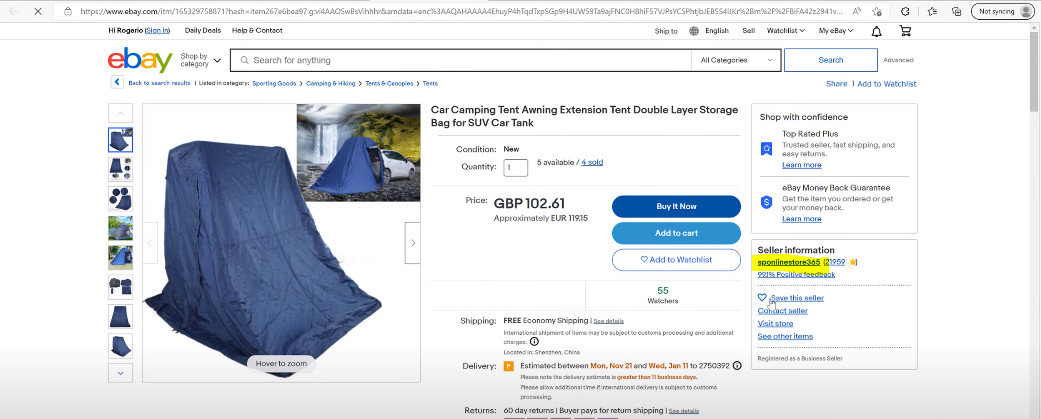The image is a screen capture from the eBay shopping site, taken on a desktop computer. The eBay webpage features a pale off-white background. Positioned in the upper right corner is the distinctive eBay logo displaying its signature colors: red, blue, yellow, and green. On the left side of the screen, there is a main image of a tent set against a white background. Accompanying this primary image, in the upper right corner, is a smaller inset photo depicting the same blue tent alongside a white SUV. Central to the screen capture are the product details, prominently written in black text. The product is titled "Car Campaign Tent, Earning Extension Tent, Double Layer Storage Bag for SUV Car Tank." Below this title, there is a small text box marked with the quantity "1" and a label for quantity to its left. Directly beneath, the price of the item is displayed, noted as £102.61 GBP (Great British Pounds).